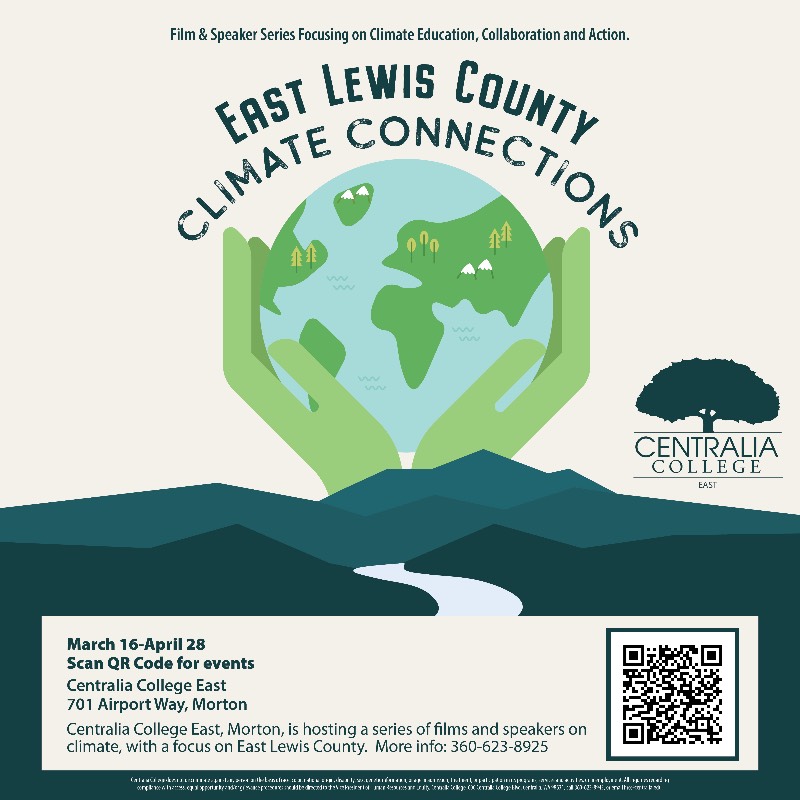The image is an advertisement for a film and speaker series focused on climate education, collaboration, and action, hosted by Centralia College East. At the top, text in an arch reads "East Lewis County Climate Connections" in black. Below this, an illustration depicts the planet Earth, represented by a blue circle with green continents, being cradled by two green hands. Beneath the hands, the landscape transitions into rolling hills in shades of blue, possibly depicting a river running through them. On the right side of the image, a white silhouette of a tree with the words "Centralia College East" is displayed. At the bottom, a white section provides event details, stating "March 16 to April 28" and "Scan QR code for events" followed by the address "701 Airport Way, Morton." A QR code is also visible in a square on the right side.